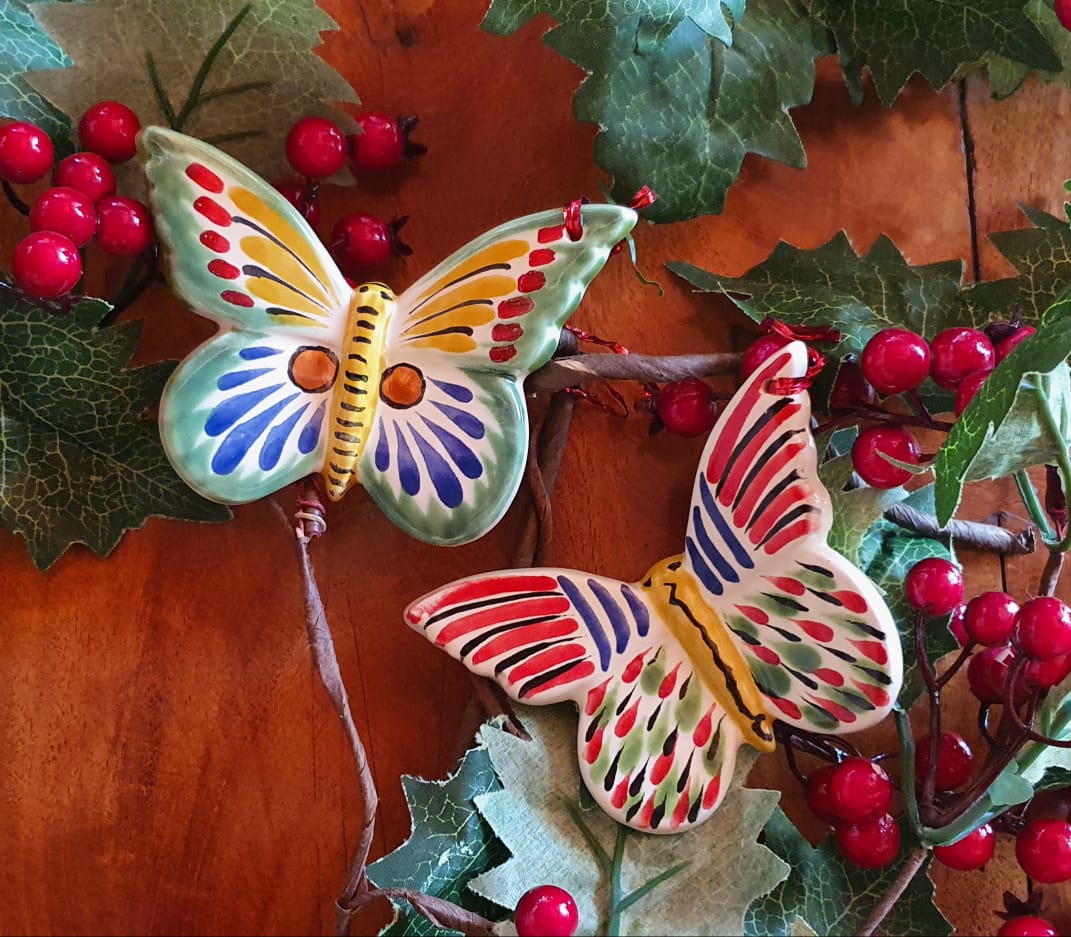This indoor daytime photograph showcases a brightly lit mid-dark stained wooden table, possibly in a kitchen. The table is adorned with artificial holly leaves and red berries, arranged like a wreath. Situated prominently on the table are two multicolored ceramic butterflies resting atop the faux foliage. The butterfly on the top left features an outline of green with accents of yellow, blue, and red, with a predominantly white bottom wing accented by black and white stripes, blue bands, and a pattern of red, green, and black droplet-like designs. The second butterfly, positioned in the bottom right, is characterized by mint green, red, and yellow hues on its upper wings and mint green, blue, and orange circles on its lower wings. Both butterflies have distinctive yellow bodies, adding to the vivid and intricate design.